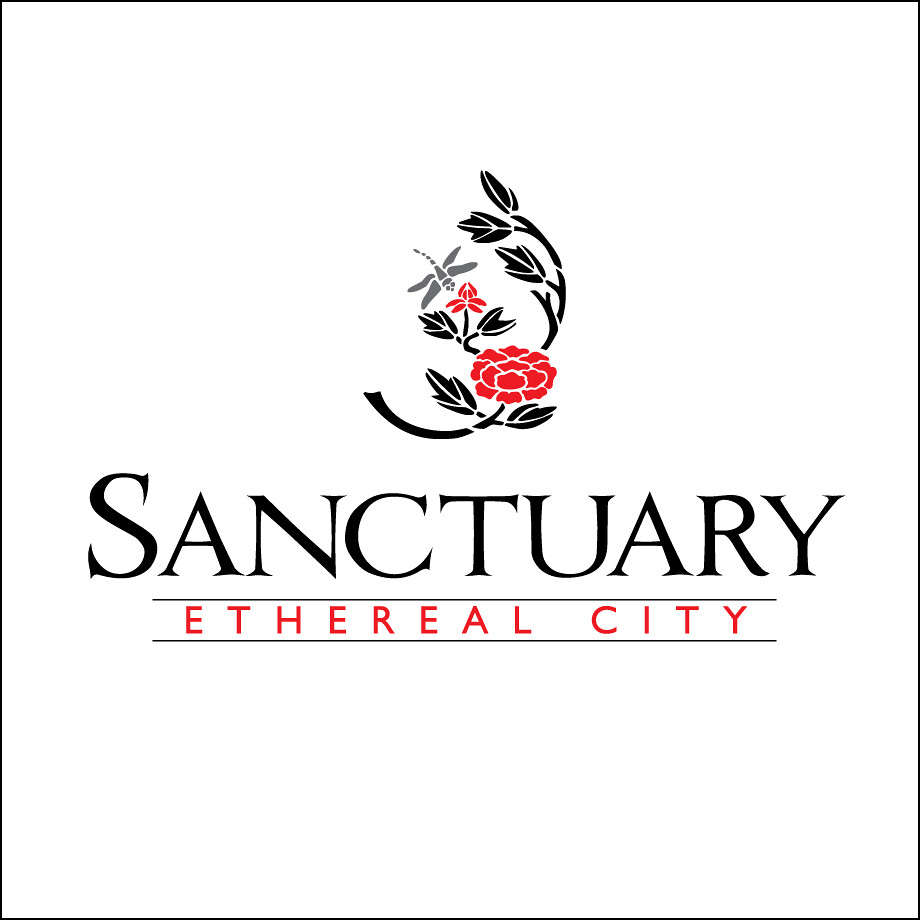The simplistic yet striking logo for the sanctuary, "Ethereal City," features a white square backdrop framed by a black border. Central to the design is a black stem with black leaves accented by delicate white lines, culminating in a prominent red poppy-like flower with numerous petals. Adjacent to the primary bloom is a smaller red flower, not yet fully open. Adding to the natural theme, a grey dragonfly is depicted flying towards the flowers. Beneath this botanical illustration, the word "Sanctuary" is prominently displayed in bold black letters. Directly below "Sanctuary," and divided by a thin grey line, the text "Ethereal City" appears in bold red lettering, framed above and below by grey lines, encapsulating the sanctuary's name within a sophisticated and cohesive design.